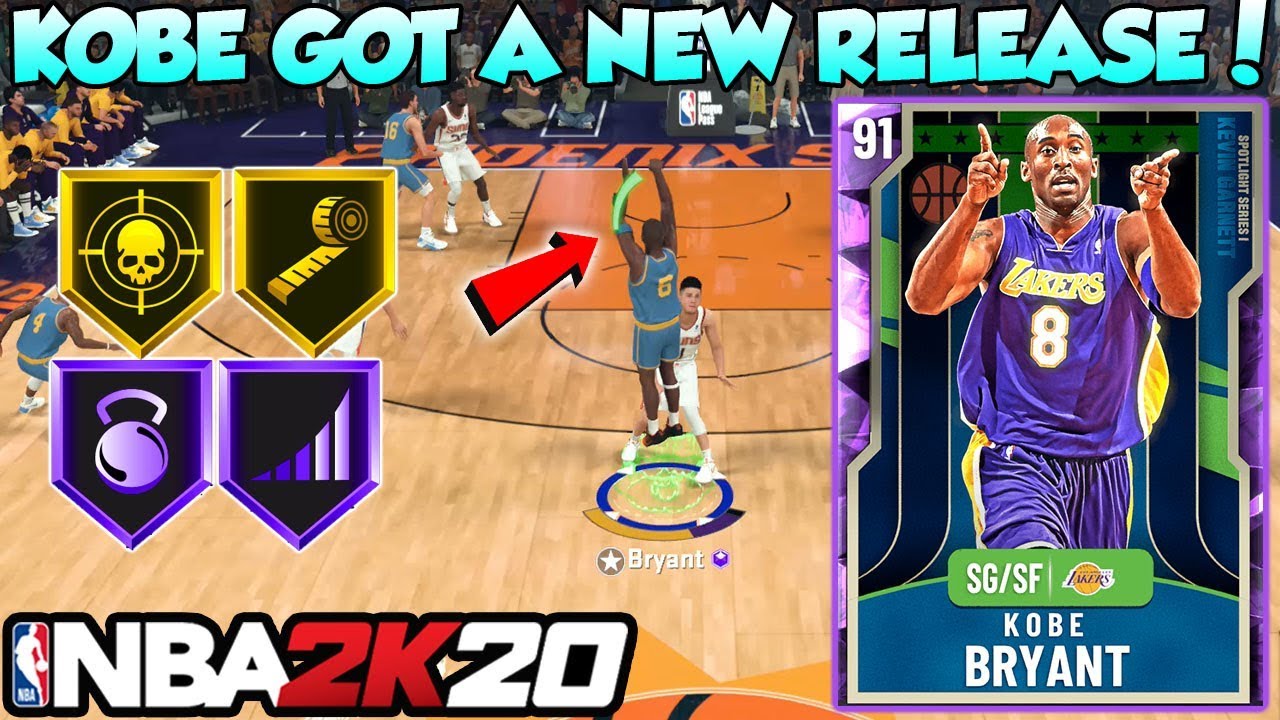This is a detailed caption for an image that is a composite screenshot from the NBA 2K20 video game. In the background, it shows in-game graphics portraying an African-American player executing a jump on a basketball court, surrounded by other virtual NBA players. At the top of the screenshot, vibrant sky-blue bubble letters proclaim, "Kobe got a new release!" A prominent red arrow points towards the jumping player, highlighting him. Adjacent to the arrow are four shield-shaped icons, arranged in a 2x2 grid on the left side of the screen. The top left shield displays a skull, the top right features a measuring tape, the bottom left bears a kettlebell icon, and the bottom right depicts an icon resembling the Wi-Fi signal. The combination of these elements suggests an update or new feature in the game related to Kobe Bryant.